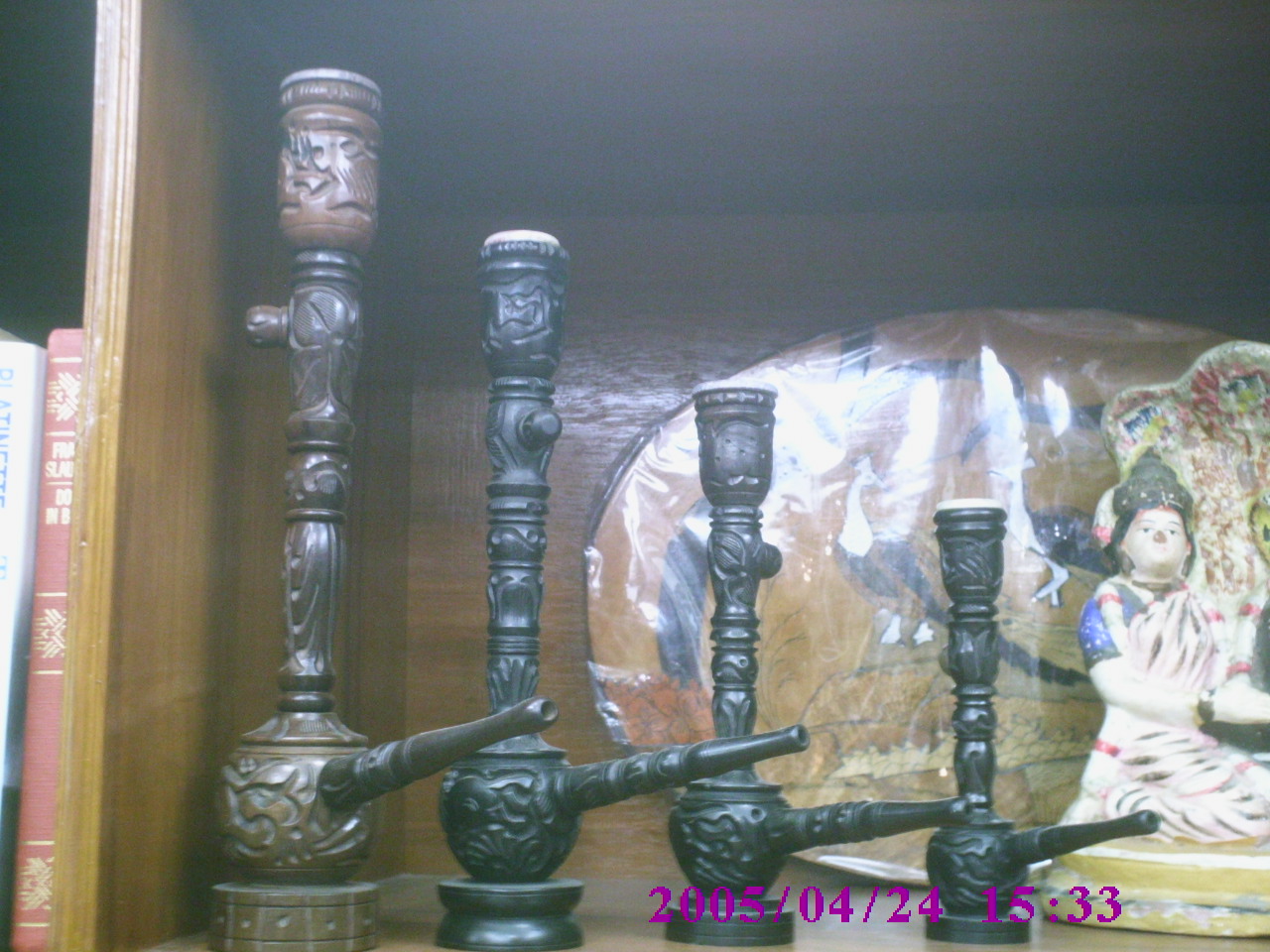This close-up photograph captures a section of a medium-colored wooden bookshelf. The main focus is on four highly ornate hookah pipes with a metallic sheen, though some might be carved from wood. These pipes feature intricate engravings and designs. The leftmost pipe is brown, while the other three are black. Each pipe tapers from a round, carved base to a tall tube, ending in what appears to be a small bowl at the top, presumably for holding smoking material. Beside the pipes, there is a handmade clay or porcelain statue, possibly a deity.

In the background, partially obscured by plastic wrapping, is an oval plaque with a delicate painting of a lady and some peacocks, adding an oriental flair to the scene. A vertical divider splits the shelf, with the left section displaying two books—a white one and a red one with only their spines visible. A garish purple watermark at the bottom right corner marks the date and time as "2005/04/24 15:33".